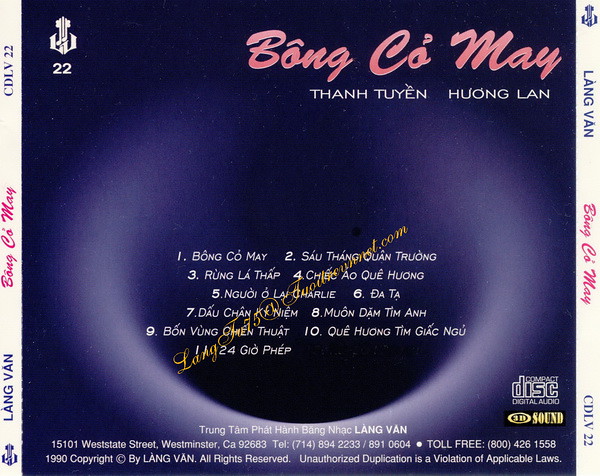The image depicts what appears to be the cover of a CD or album. Dominating the center is a large purplish square backdrop, where song titles are listed, numbered sequentially from 1 to 11. The titles are written in a language that is not easily recognizable. The overall color scheme includes tan, purple, pink, white, black, gray, and yellow, blending harmoniously throughout the design. 

On the left, the name "Lang Van" appears, presented in a white rectangle with purple text. Towards the top, additional text reads "Bong Kho Mae," "Thanh Tuyen," and "Hong Lan," possibly indicating either the album title or the names of the artists involved. A stylized script in pink features prominently, presumably the album's title "Mon-Ko-Mei." The intricate design and use of colors suggest an artistic and carefully crafted album cover, possibly indicating its content is related to music. The mixture of language elements and the visual style make it a striking and evocative image.